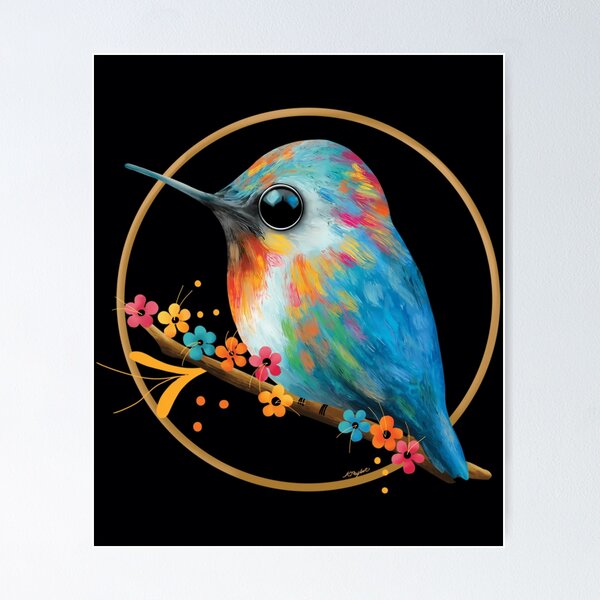This captivating image, set against a stark black background, features a mesmerizing painting or AI-generated depiction of a small, plump bird that appears both vibrant and imaginative. The bird is perched delicately on a brown branch adorned with colorful flowers arranged in a sequence from left to right: pink, yellow, blue, orange, pink, yellow, blue, and orange. Adjacent to these flowers are yellow sprouting leaves and various orange and yellow dots adding to the vivid composition. The bird itself is enveloped within a gold circle that frames most of its body, with only its slender beak and part of its tail protruding beyond.

The bird showcases an array of stunning hues: primarily a royal blue with bright variations across its body, featuring splashes of hot pink, gold, fluorescent green, and white. Its beak is a light blue shade, transitioning to a blend of black, gold, orange, and red under the beak and at the back of its head. The bird's chest is downy white, and its wings are primarily blue. Additionally, there is a distinct orange marking on its forehead. A prominent feature of the bird is its enormous, dilated black eye that adds an eccentric and captivating focal point to its overall appearance. The scene is signed within the gold circle, though the signature remains illegible. The entire composition is encapsulated within a square format, emphasizing the contrast between the vibrant subjects and the dark background.